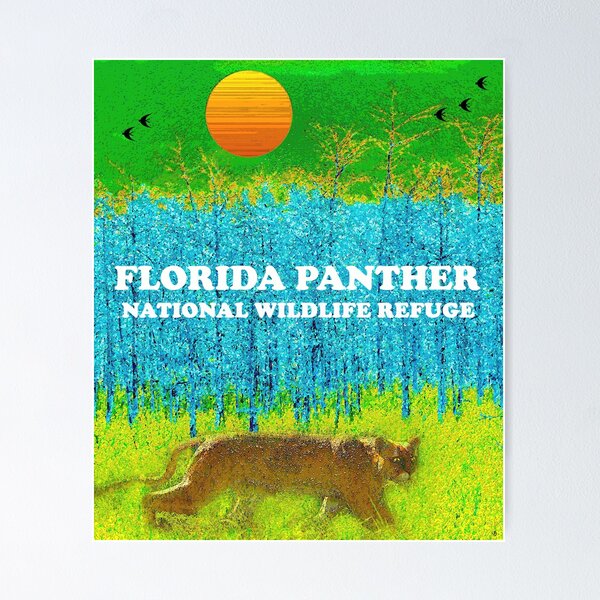The image appears on a vibrant book cover or poster, likely related to the Florida Panther National Wildlife Refuge. At the top, it depicts a striking green sky with a yellow and orange striped sun positioned slightly to the left. Scattered across the sky are several black birds, all facing left. Below this, the landscape transitions into a field of light green grass, above which stand large trees in a bright teal blue color, with darker blue trees interspersed among them. In the center of the field, a large, tan cougar is seen trotting to the right. Bold white text reading "Florida Panther National Wildlife Refuge" is prominently displayed in the middle of the image, nestled within the trees. The overall design is highly colorful and dynamic, utilizing green, blue, yellow, orange, and red hues to create a visually striking effect.